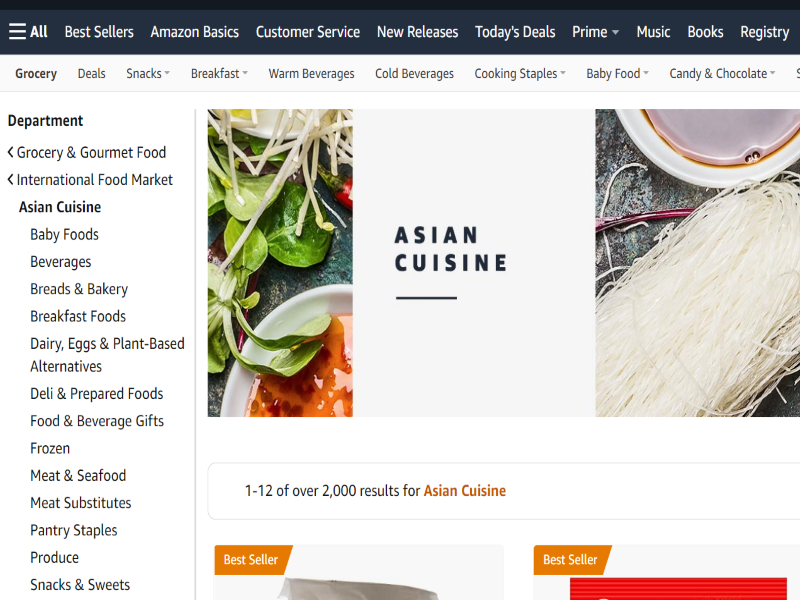The screenshot displays a section of the Amazon website, identifiable by its signature layout and design elements. At the top of the screen is a solid black navigation bar featuring a menu icon (three horizontal lines) followed by the word "All." Next to this, several tabs are visible, including "Bestsellers," "Amazon Basics," "Customer Service," "New Releases," "Today's Deals," "Prime," "Music," "Books," and "Registry."

Just below this main navigation bar, there are specific category options listed: "Grocery," "Deals," "Snacks," "Breakfast," "Warm Beverages," "Cold Beverages," "Cooking Staples," "Baby Food," "Candy," and "Chocolate." In this screenshot, the "Grocery" option has been selected.

On the left side of the screen, a sidebar displays different departments, and "Asian Cuisine," which is located under the "International Food Market" category, has been chosen. The main section of the screen shows an image depicting Asian food—specifically a white bowl filled with what appears to be chicken in a brown sauce accompanied by white rice noodles on the far right.

Centrally located on the screen is a white rectangle that reads "Asian Cuisine." Below this, a banner indicates "1-12 of over 2,000 results for Asian Cuisine." Additionally, two product images partially appear at the bottom of the screen. Both are marked with an orange "Bestseller" tag in the top left corner. The product on the left contains a white object, while the one on the right features a red object.